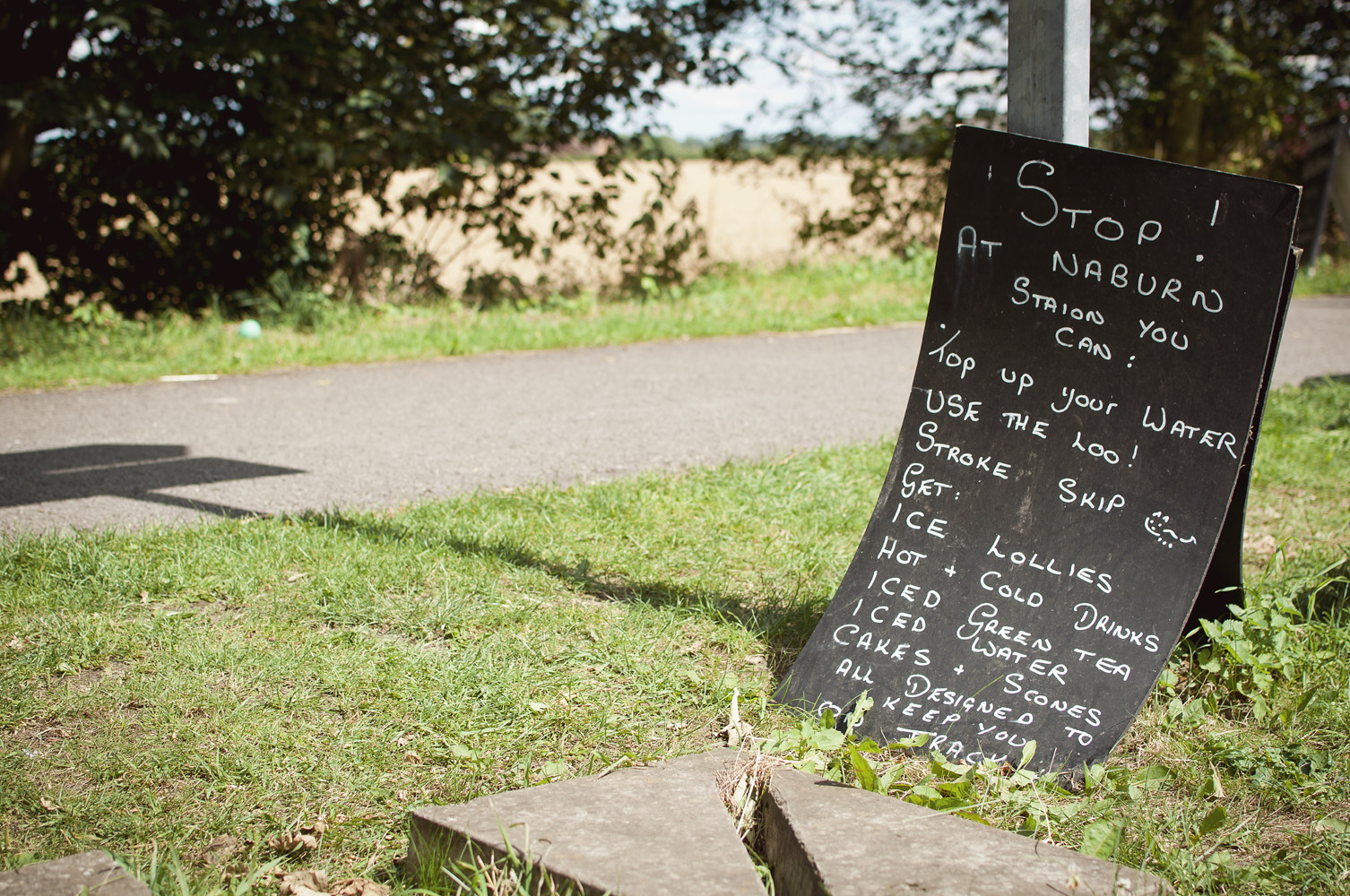In this outdoor color photograph, a sign leans against a white metal post beside a paved path, amidst a grassy area. The black wooden sign, featuring white handwritten text, appears slightly bent and is partially propped up on the ground. The text reads: "Stop at Naburn Station; top up your water, use the loo, get ice lollies, hot and cold drinks, iced green tea, iced water, cakes, and scones, all designed to keep you on track." The foreground reveals two triangular pieces of concrete and a concrete platform surrounded by grass. Beyond the sign is a narrow strip of grass, trees, and a brown field, under a clear blue sky.